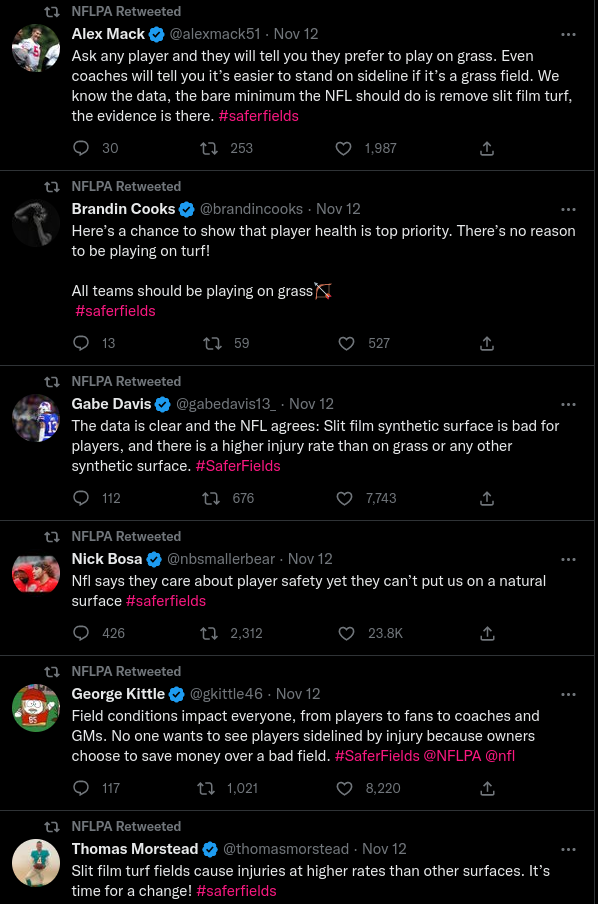The image is a screenshot displaying a Twitter conversation on a jet-black background. The screenshot features six different posts, arranged from top to bottom, each separated by a thin gray line. The names of the posters, in order from top to bottom, are Alex Mack, Brandon Cooks, Gabe Davis, Nick Bosa, George Kittle, and Thomas Morstead. Each poster has a blue verification checkmark next to their name and a profile picture in a circular frame to the left of their name, with some pictures featuring football players.

The date of the tweets is November 12th. The conversation begins with a tweet from Alex Mack, who states, "Ask any player and they will tell you they prefer to play on grass. Even coaches will tell you it's easier to stand on the sideline if it's a grass field. We know the data. The bare minimum the NFL should do is remove slit film turf. The evidence is there." 

Following Mack's tweet, other notable players like Brandon Cooks, Gabe Davis, Nick Bosa, George Kittle, and Thomas Morstead engage in a discussion emphasizing the preference for grass fields over artificial turf. Throughout the image, red hashtag links with the text "#SaferFields" are visible, as well as tags "@NFLPA" and "@NFL."